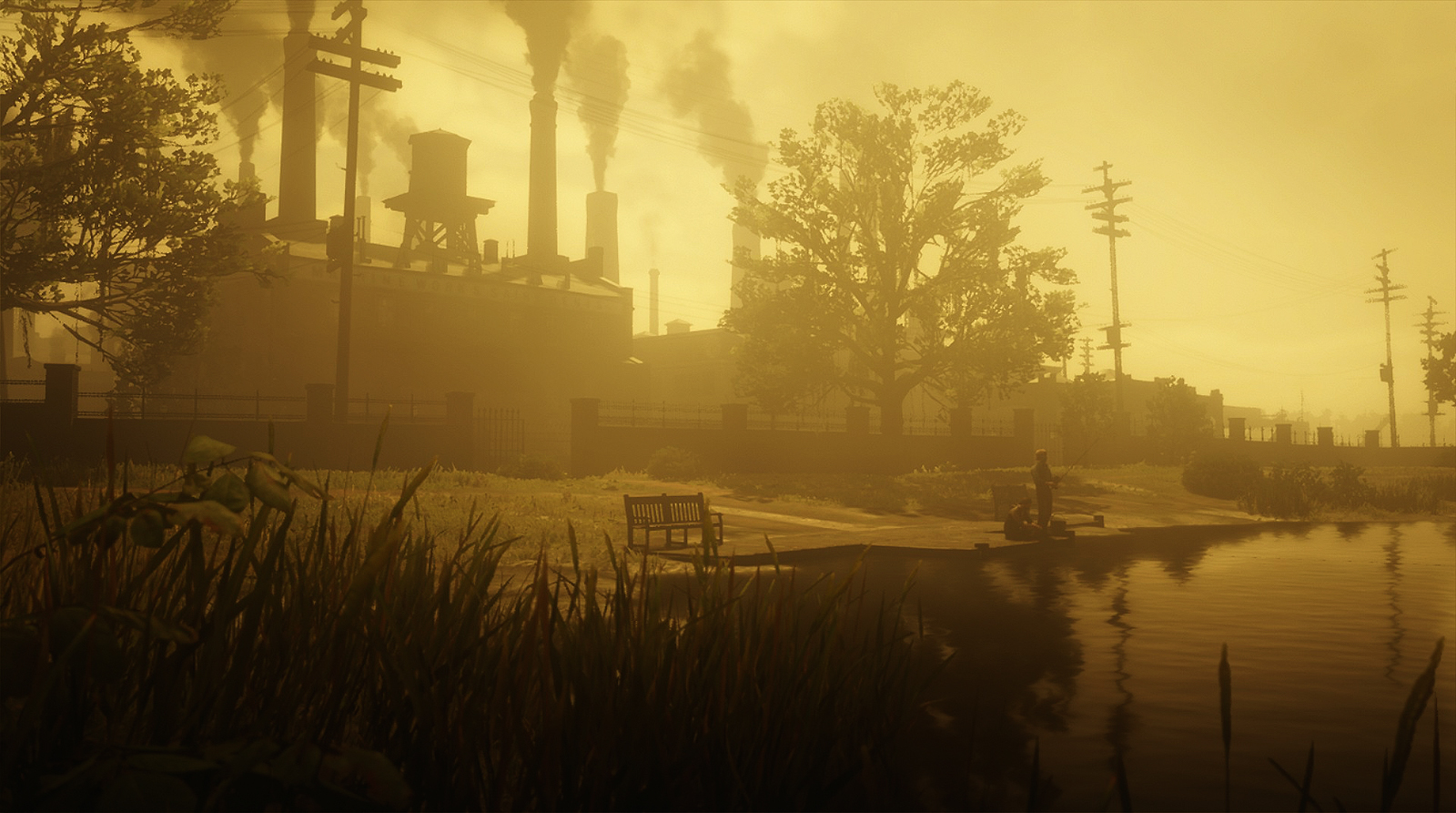A sepia-toned photograph, dominated by yellow hues, captures a tranquil yet industrial scene. In the lower left corner, tall grass extends halfway into the center of the image, where it meets a river adorned with cattails on the right side. Across the river, two small, indistinct figures—possibly fishing or merely standing—are positioned, with one sitting and the other standing amidst a few unidentifiable objects. Nearby, a structure that could be either a wooden dock or a cement platform, given the challenging color scheme, features a wooden bench at its edge.

The platform seems to conclude a path that descends a gentle slope to the river's edge. A fence with cement blocks and a higher, metal railing contains the riverbank and the hill, marking a boundary between natural elements and a heavily industrial backdrop. Smokestack emissions from a nearby factory billow into the sky, flanked by power lines, juxtaposing the serene riverside nature with the stark, imposing industrial landscape of the town.